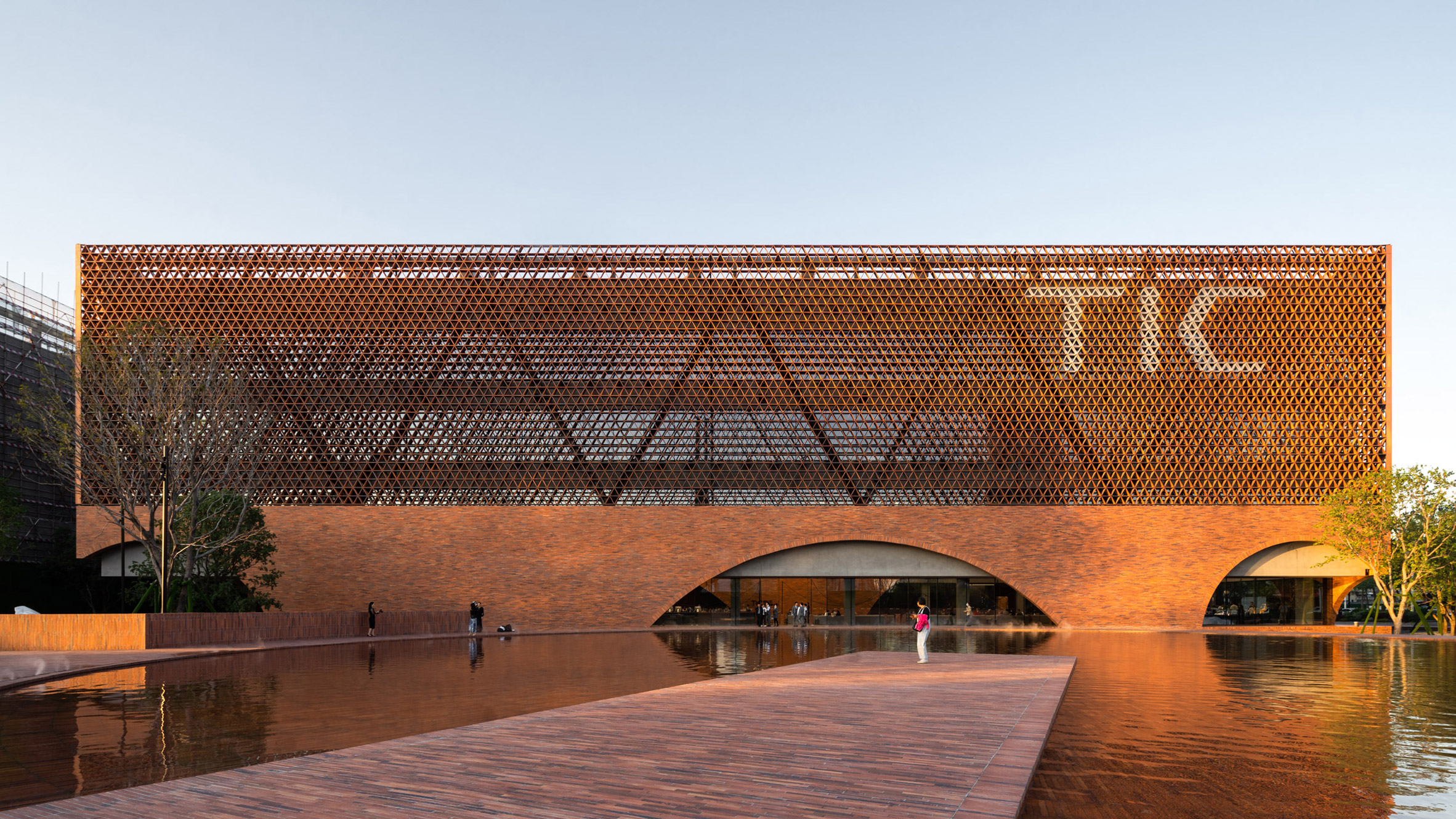The photograph features a contemporary office building constructed primarily of a rustic brick color, symbolizing vernacular building methods. The structure stands tall with a large rectangular form and prominently displays the large white letters "T.I.C" on a screen-like mesh at its top, offering a see-through view to the other side. The base of the building showcases two arches with glass windows and doors, acting as entrances. Surrounding the building is a water feature, appearing to be a man-made lake or pond, with a brick walkway extending halfway into the water, providing access to the building. This walkway is flanked by trees on either side, adding to the aesthetic appeal. The sky overhead is a vivid blue, indicative of late afternoon light. Individuals can be seen near the entrance and scattered around the building's exterior, suggesting it is a bustling location at this time of day.